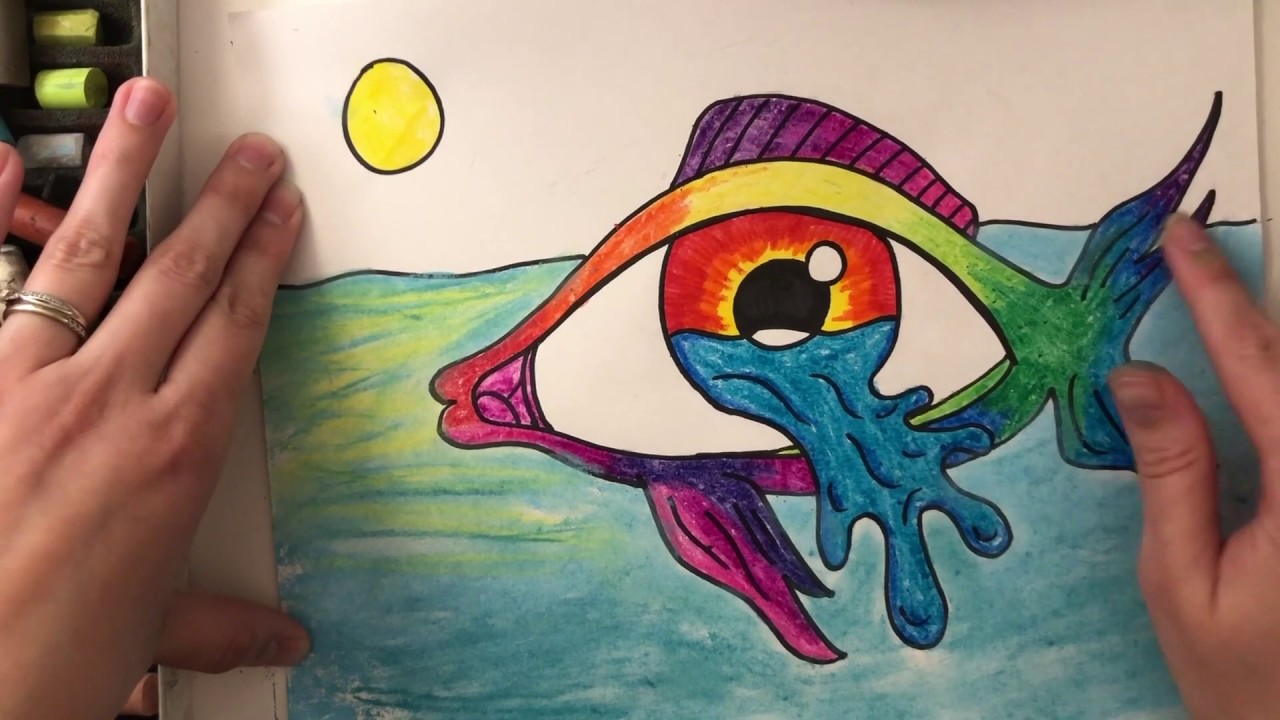The photograph showcases a vibrant, crayon-colored artwork being held up by two hands, one of which has a ring on the ring finger. The artwork, likely created by a child or an adolescent, features a colorful, cartoon-like fish partially submerged in water. The fish displays an array of colors including orange, red, green, yellow, magenta, purple, and blue, with distinct purple and blue fins. Notably, the fish has a large, human-like eye, which is yellow and orange and spills out blue tears that resemble waves. Above the fish, a bright yellow sun is positioned in the top left corner, adding a touch of warmth to the aquatic scene. The picture is held over a table with some chalks visible to the left, and appears to be inside a box of some sort, combining elements of land, sky, and ocean into a whimsical, imaginative composition.